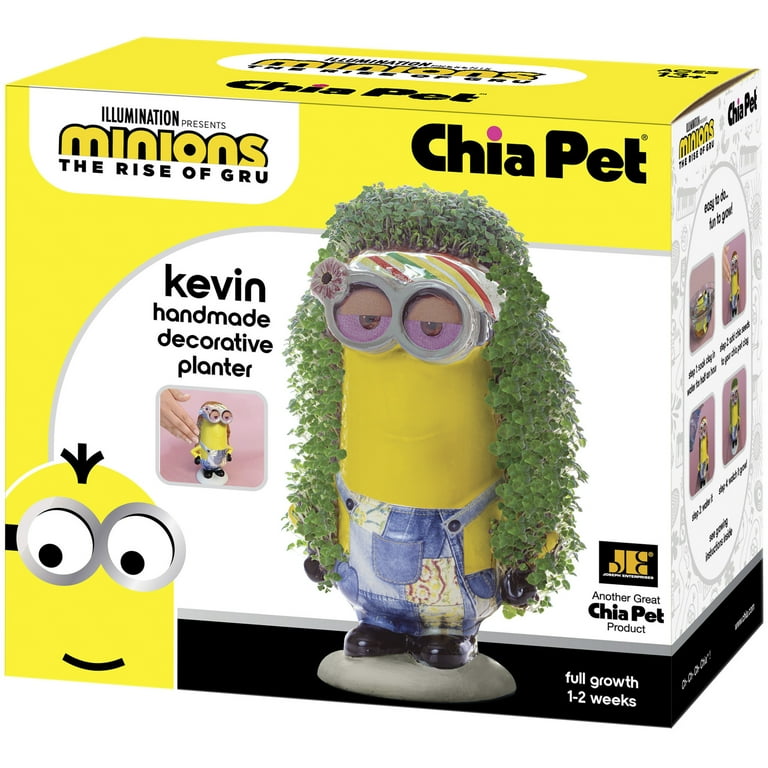This image showcases a box for a Chia Pet product, specifically a collaboration with Illumination Studios' "Minions: The Rise of Gru." The predominantly yellow box features a white section in the upper left that reads "Illumination presents Minions: The Rise of Gru," with the Chia Pet logo on the upper right. Central to the box is an image of the fully grown Chia Pet, depicting a Minion named Kevin. Kevin, wearing denim overalls, dark black shoes, and goggles that resemble floral designs, has vibrant green plant matter sprouting from his head and cascading down to mimic long hair. To the left of this image, text reads "Kevin Handmade Decorative Planter," beside a smaller illustration of Kevin sans chia growth. The box also mentions "Full Growth in One to Two Weeks" and highlights this as "Another Great Chia Pet Product." Additionally, instructions and imagery on the side convey the easy and fun process of nurturing the Chia Pet.